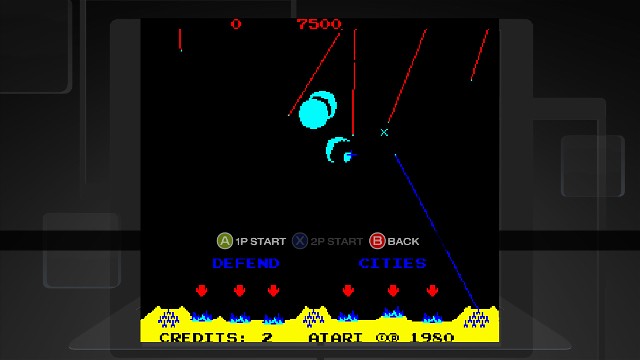This is a color image depicting a vintage video game screen, reminiscent of an early Atari game. The background features interlocking squares in various shades of gray, creating a tiled effect that fades into black towards both the left and right edges of the screen. Dominating the center is a prominent black square, topped with the numeral "7599" in bold red. Descending from the top of the image, a series of red lines can be seen, converging towards the middle, where light blue circles hover. Additionally, a singular blue line extends upward from the bottom.

On the left side of the screen, a list of player scores is displayed. Adjacent to this text is a green circle, mirrored by a red circle on the right. Directly below these, the words "DEFEND" and "CITIES" are printed, each aligned under their respective circles. A sequence of small, red arrows is positioned beneath these words, adding to the graphical elements.

The bottom portion of the screen is segmented by a yellow layer interspersed with blue sections. Printed in black text within this area is a credit line that reads, "Credits to Atari," followed by a list of numbers that are not clearly legible.